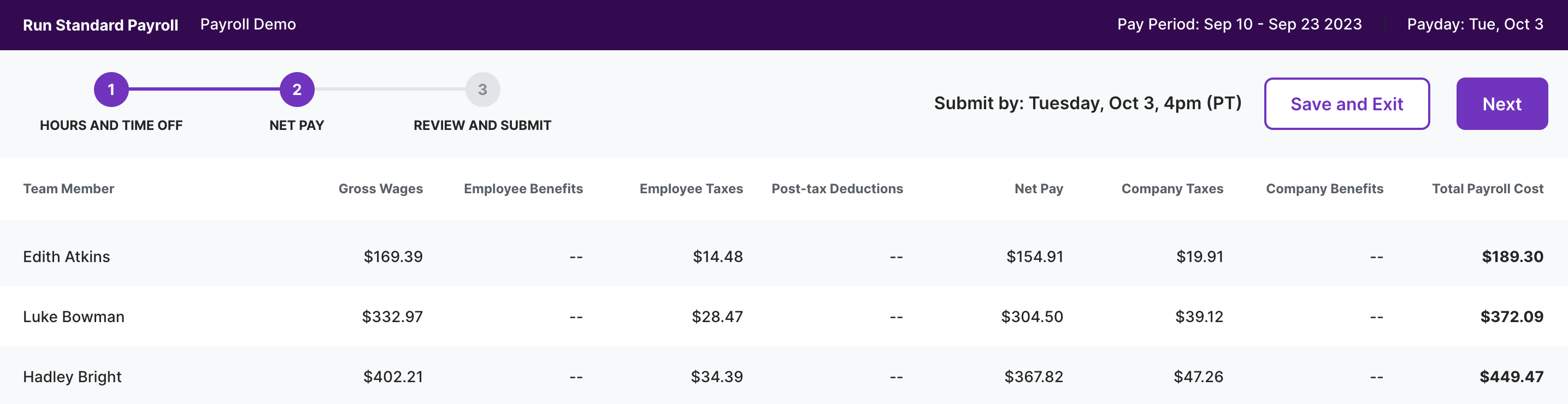The image depicts a computer screen displaying a payroll management interface. In the upper left corner, the words "Run Standard Payroll" are prominently displayed, followed by "Payroll Demo" indicating a demonstration mode. A deep purple rectangle stretches across the top, primarily empty except towards the right-hand side where it lists critical payroll period details. It specifies the pay period as "September 10th to September 23rd, 2023" and marks the payday as "Tuesday, October 3rd."

Beneath this section, there is a sequential guide for processing payroll, marked by three numbered purple circles connected by a line. The first step, labeled "1," is "Hours and Time Off," followed by step "2," "Net Pay," and finally, step "3," "Review and Submit."

Below these instructions is a detailed spreadsheet-like area, which includes columns for various payroll components. The headers from left to right are: "Team Member," "Gross Wages," "Employee Benefits," "Employee Taxes," "Post-Tax Deduction," "Net Pay," "Company Taxes," "Company Benefits," and "Total Payroll Costs." This organized layout is likely filled with rows of team member data, summarizing the financial breakdown of each employee’s payroll.

Overall, the screenshot provides a comprehensive view of the payroll process, illustrated with a clear step-by-step guide and detailed employee financial data categories.